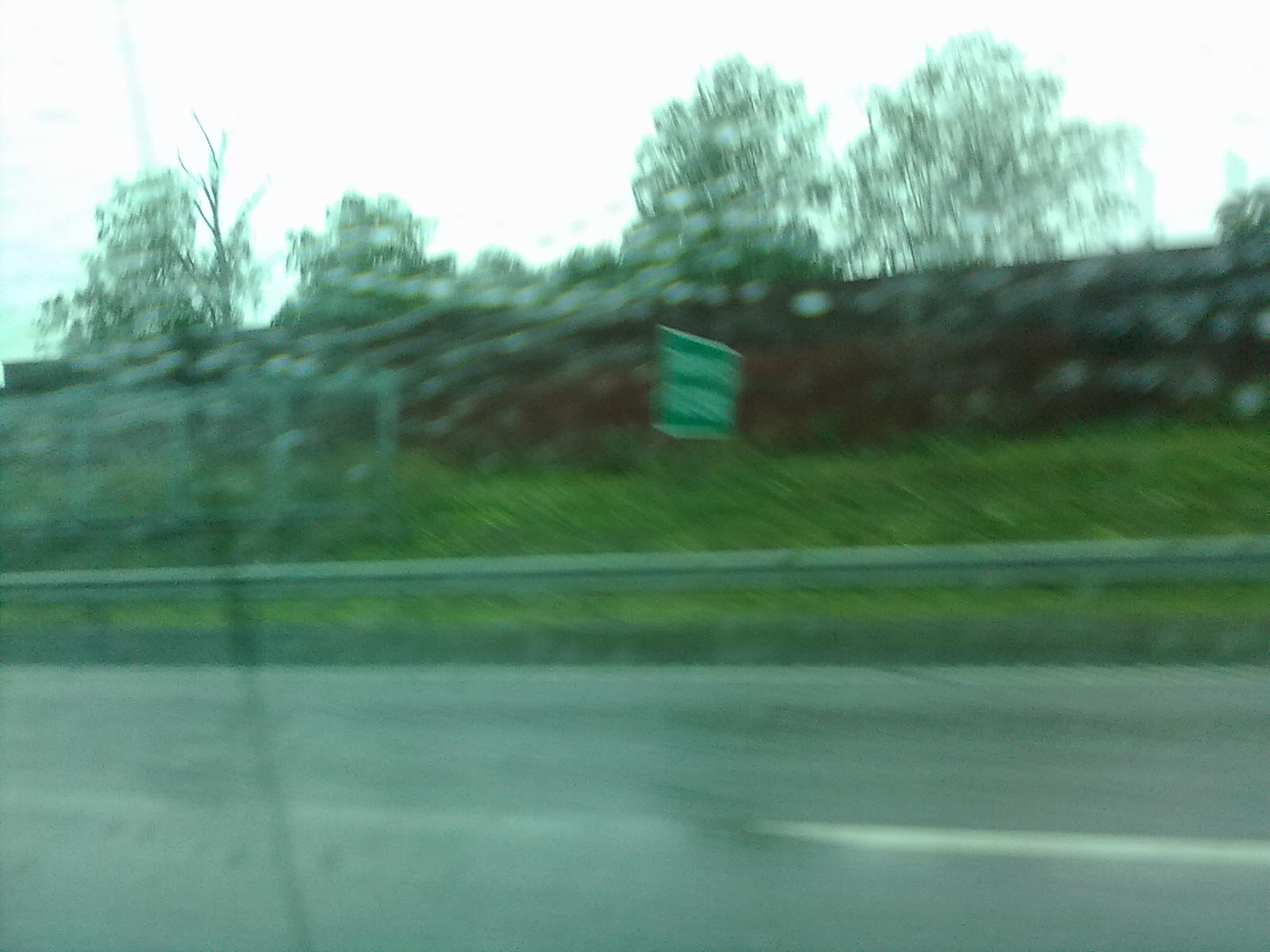A rainy day view captured from the inside of a moving car, showing droplets of rain and window glare on the side window. Outside, a blurred green roadside sign with unreadable white text stands behind a steel guardrail which separates the road from a grassy incline. The sign is positioned two lanes away from the viewer's car, on a clear stretch of road. In the background to the right, a rocky mound is visible with the tops of trees emerging against a backdrop of a grey, overcast sky. The overall image is blurry, emphasizing the movement and the wet conditions.